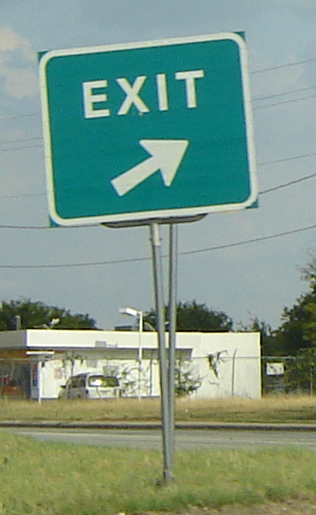This image captures a close-up of a green exit sign, prominently displayed on a metal pole standing approximately four to five feet tall. The sign features a distinct white outline and the word "EXIT" in green text, accompanied by an arrow pointing diagonally upward to the right. The base of the pole is embedded in a grassy patch, which seamlessly transitions into a road visible behind the sign. On the far side of the road, another stretch of grass appears, leading up to a white building surrounded by a six-foot-high metal mesh fence. A silver car is parked in front of the building, while trees form a picturesque backdrop. The sky above is mostly clear with a few wispy clouds, providing a serene blue canvas. Power lines stretch horizontally across the scene, adding a subtle layer of depth to the composition.